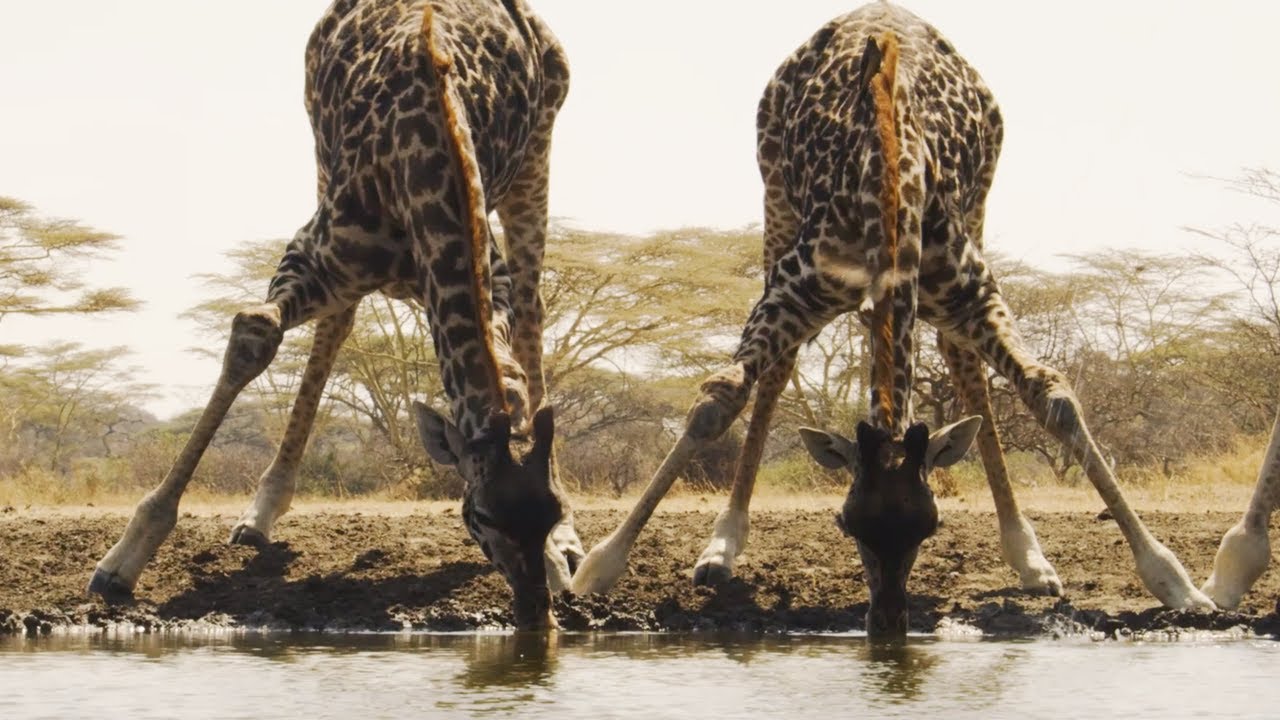The image depicts two giraffes in an ungainly, yet graceful stance at a watering hole in Africa, their long necks stretched down towards the water. Both giraffes have their front and back legs splayed wide apart to facilitate drinking, displaying their tawny coats adorned with irregular brown spots. The giraffes' two horns and cute, expressive ears are visible, along with a hint of a reddish mane. To the right edge of the photograph, the hoof of a third giraffe can be seen. The scene is set in their native habitat, with a backdrop of green, bonsai-shaped acacia trees and scrubby, muted grasses. The distant hills and a grayish white sky complete the serene landscape shot from the opposite bank, capturing the essence of this tranquil moment in the wild.